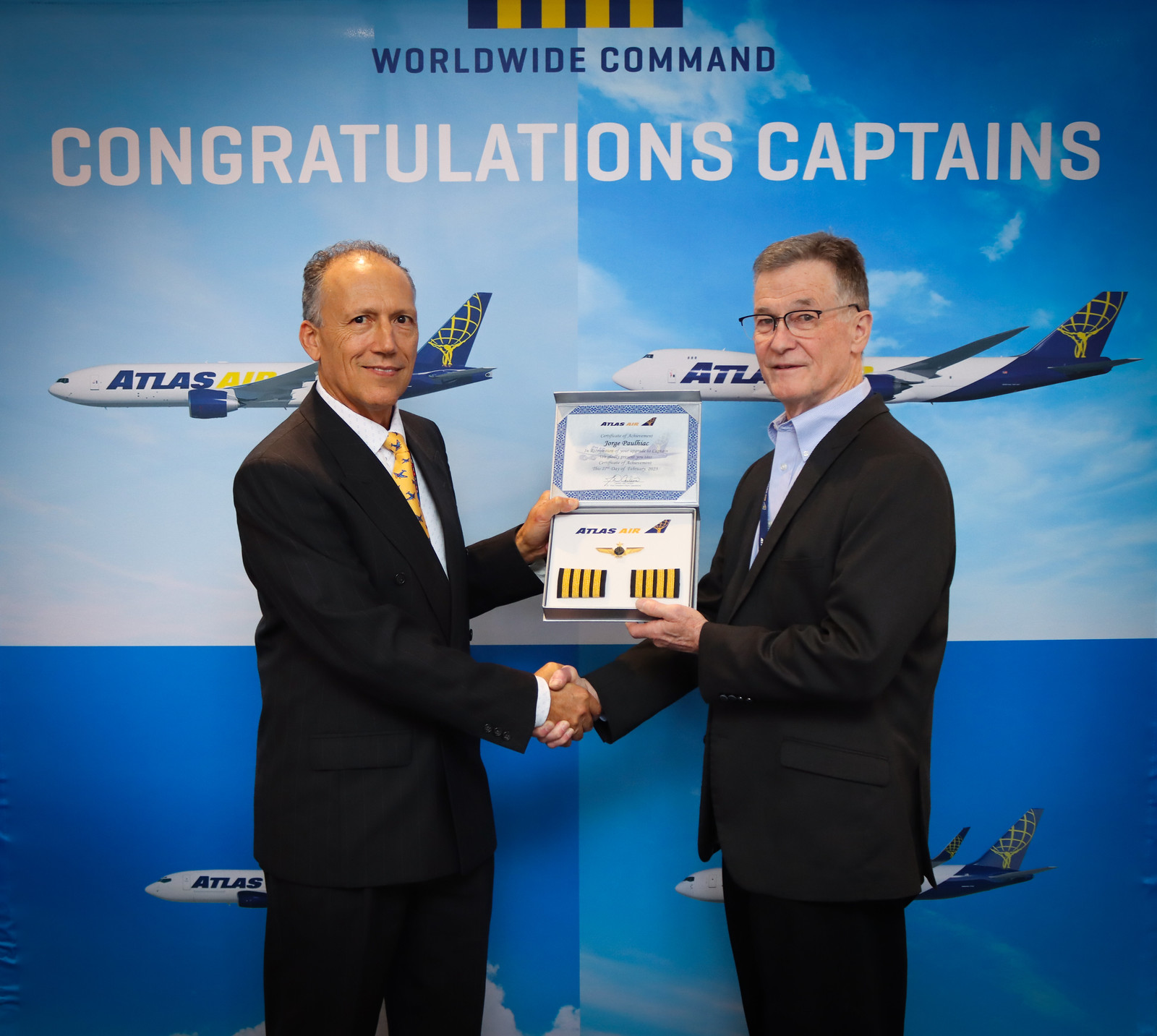In this image taken at an award ceremony, two older men in black suits are standing side by side, shaking hands while jointly holding an open certificate case. The man on the left, who has grey balding hair and is dressed in a white shirt with a yellow tie featuring airplanes, appears to be presenting the certificate. The man on the right, who wears glasses, has short brown hair, and is dressed in a white shirt without a tie, can be identified as Jorge Paulyac, as his name is visible on the certificate. The award case also contains a medal with airplane wings. They stand in front of a striking backdrop divided into four sections, each depicting different skies with Atlas Air jets. The top of the backdrop has a banner with blue and white vertical stripes. Below this banner, bold blue text reads "Worldwide Command," and beneath it, in larger white capital letters, it says "Congratulations Captains!" The overall atmosphere is one of professional recognition and celebration, with both men looking happy yet serious.